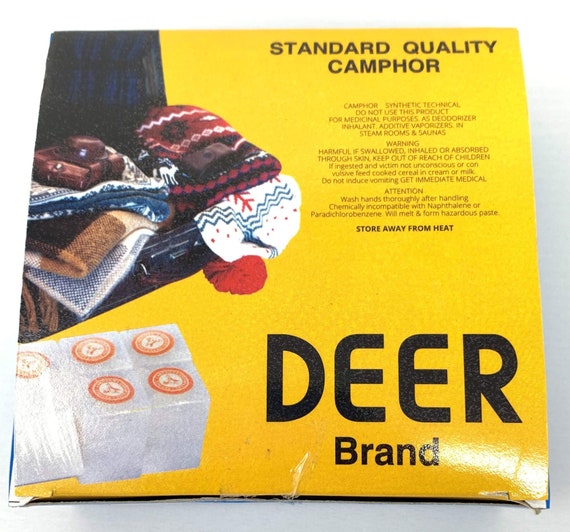The image depicts the packaging of a Deer Brand standard quality synthetic camphor product. The packaging is a bright yellow color featuring prominent black letters that state "Deer Brand" and "Standard Quality Camphor". The top of the package carries extensive warnings advising against the use of the product for medicinal purposes, including as a deodorizer, inhalant, or additive in vaporizers, steam rooms, and saunas. The warnings highlight the hazardous nature of the camphor, detailing the potential harm if swallowed, inhaled, or absorbed through the skin, and giving clear instructions on handling and emergency response in the event of ingestion. Additionally, the packaging depicts images of winter clothing items like woolen caps, scarves, and fleecy materials in colors such as white, red, and brown. The lower segments of the packaging show white cubes of camphor. There are also cautionary notes about the chemical incompatibility of camphor with naphthalene or para-chlorobenzene, noting that such mixtures will melt and form a hazardous paste. Overall, the packaging is informative and visually detailed, communicating both the brand’s identity and extensive safety warnings.